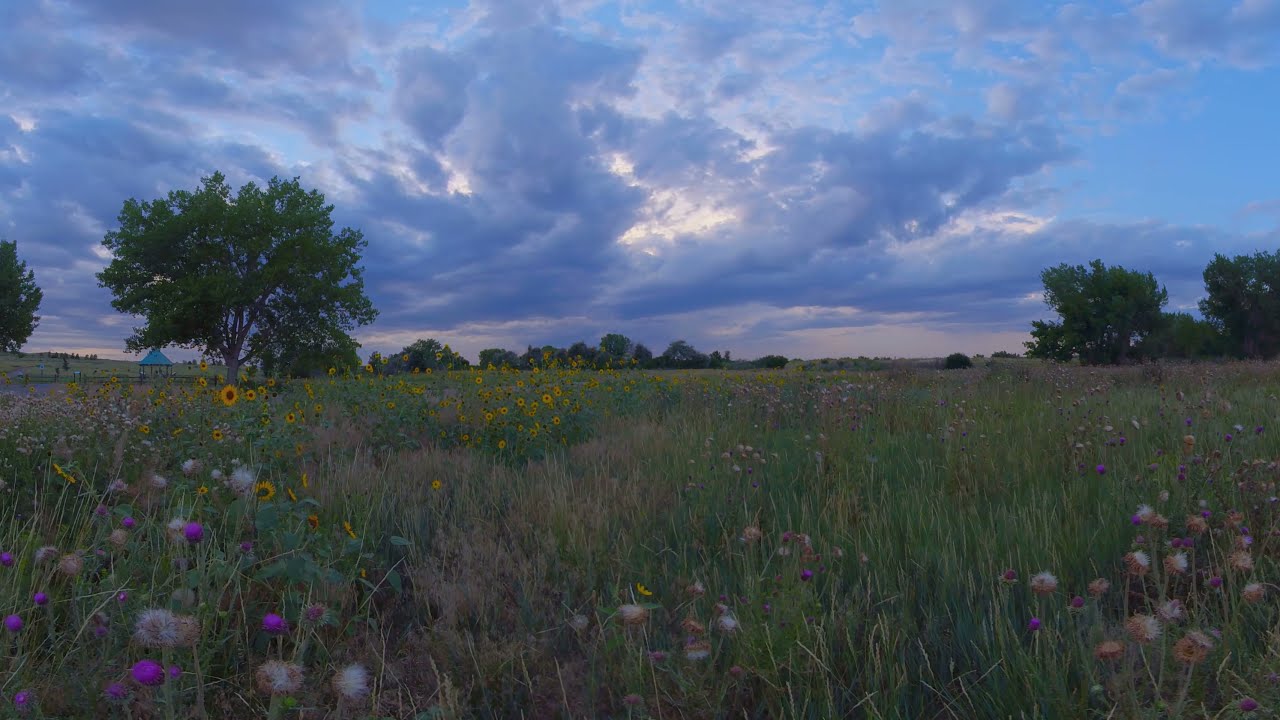The image captures a serene, deserted field teeming with a variety of wildflowers and tall, unkempt grass. Prominent among the flowers are yellow sunflowers and white dandelion puffs, with occasional hints of other blooms like brown flowers resembling black-eyed Susans and purple-topped clovers. The left side of the field features a striking blue tent nestled amongst larger trees, lending a touch of human element to the otherwise wild landscape. The field extends toward a backdrop of trees on both sides, framing the picturesque scene. The sky overhead is an overcast mix of thick, white, fluffy clouds and patches of blue, allowing only a muted light to filter through, casting a tranquil and dim ambiance over the expanse of flowers and greenery.